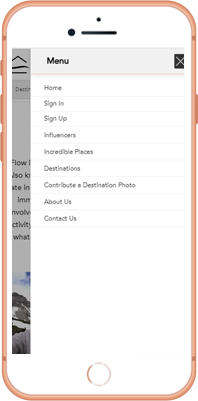This screenshot displays a segment of a web page with a prominent focus on a navigation menu. The menu heading "Menu" is highlighted in black text on a light blue bar, which features a close button ('X') on the far right. Below this bar, a list of navigation options is presented in dark blue text against a white background. These options include: "Home," "Sign In," "Sign Up," "Influencers," "Incredible Places," "Destinations," "Contribute a Destination Photo," "About Us," and "Contact Us."

To the left of this navigation menu, there is a vertical sidebar that appears partially truncated. The visible text at the top of the sidebar reads "Destination," followed by fragments of words such as "flow," "I," "KN," "ATE IN," "IMM," "NVOLV," and "WAT." These seem to abbreviate or cut off the titles of various menu items or sections.

At the bottom of this sidebar, an image is partially visible, showing what appear to be rocks against a background of either water or sky, characterized by a mix of blue and white colors.